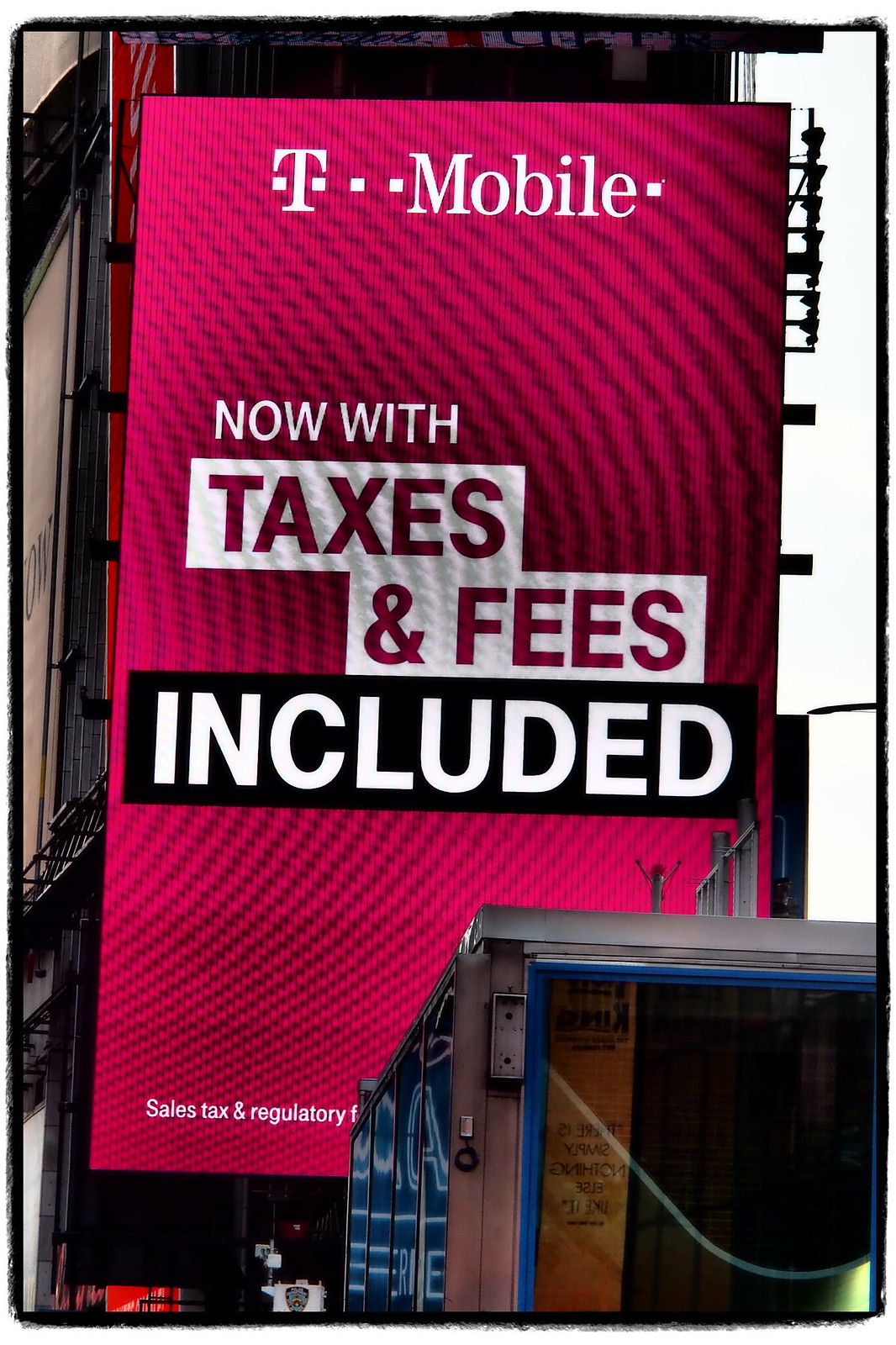This photo captures a sizable, electronically-lit T-Mobile billboard affixed to the side of a building, with a visible fire escape and partially obscured by a truck on the street. Predominantly pink with dark, circular detailing that fans out into a spiral, the billboard prominently features "T-Mobile" in white letters at the top. Right below it, "Now with Taxes and Fees Included" is displayed; "Taxes and Fees" appear in cut-out letters revealing the pink background, and "Included" is highlighted in white against a black strip, making it particularly standout. At the bottom, in smaller white text, partial words "Sales Tax and Regulatory" are visible but partially blocked by the truck, which is medium-sized and blue with a silver-edged open back. Inside the truck, a tall cardboard box can be seen. Off to the left, a small portion of another building and a different billboard is visible but partially cut off by the photo's edge.